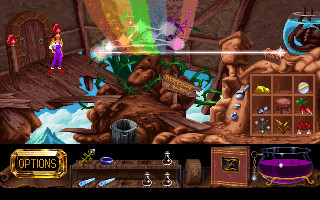This image appears to be a screenshot from a video game, depicting a busy and detailed scene. The character, dressed in purple overalls and a red hat, stands in a rustic, brown room with a closed, rounded wooden door that has a matching frame. The room is dirty, with sections of the floor missing, giving the impression that it is high up in the mountains. A plant is growing through the floor, and a rainbow is visible in the lower left-hand corner. In yellow text, the word "options" appears at the bottom left of the screen. The character's inventory is visible at the bottom, showing various potions. On the middle right, there is a book, and in the lower right corner, there is a bowl containing purple powder or sugar.